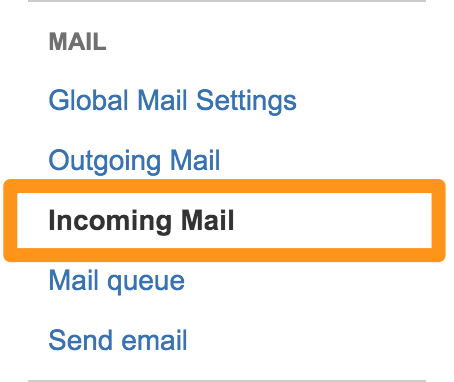This image is a screenshot of a menu from a mail application. The menu is set against a white background and is framed by two thin light gray lines, one at the top and one at the bottom. At the top of the menu, the word "MAIL" is prominently displayed in all caps, rendered in a gray font. Below this heading, there are two lines of blue text: "GLOBAL MAIL SETTINGS" and "OUTGOING MAIL." The next line of text is in bold and black, reading "INCOMING MAIL." This line is distinctly highlighted with a thick orange rectangle surrounding it. Following this are two more lines of blue text: "MAIL CUE" and "SEND EMAIL." The overall layout is mostly square in shape, with the highlighted "INCOMING MAIL" text extending slightly beyond the width defined by the thin gray lines at the top and bottom.